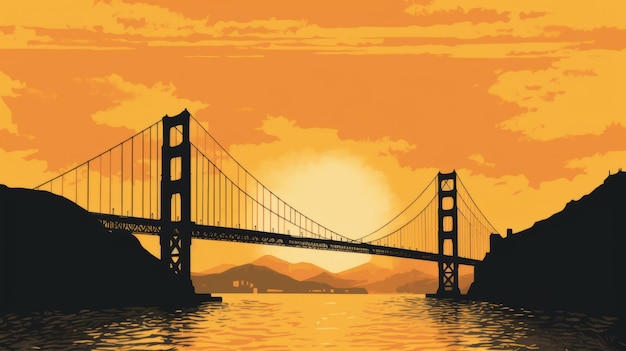The illustration depicts a dramatic silhouette of the Golden Gate Bridge against a vibrant, setting sun. From an ocean-level perspective, the viewer looks directly at the bridge, which stands starkly in black against the brightly colored sky. The sun is centered behind the bridge, casting a brilliant light that transitions from yellow at its core to various shades of orange across the horizon. This illumination gives the sky a rich gradient effect with darker orange clouds interspersed. Both the left and right sides of the bridge are flanked by silhouetted land masses, creating a sense of symmetry despite minor artistic liberties taken with the bridge's segment design. Beneath the bridge, the water of the bay reflects the sunny hues, continuing the palette of yellows and oranges. In the distance, a range of softly outlined hills completes this visually striking scene.